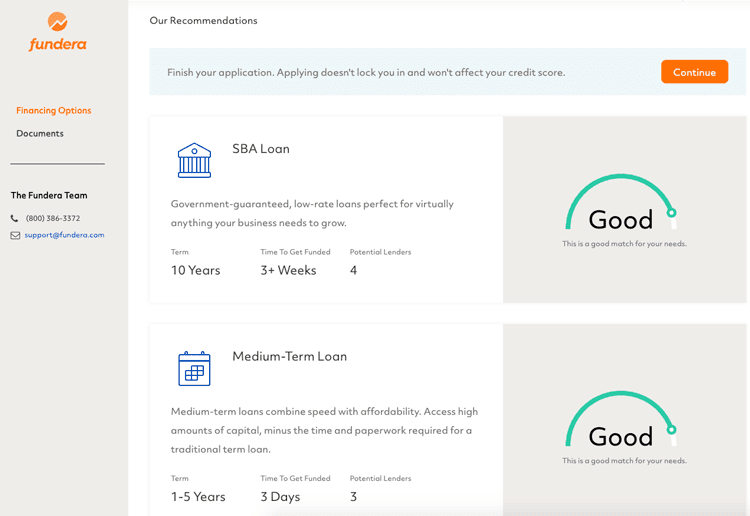The image is a screenshot of the Fandera application interface, likely taken on a desktop computer. The left section of the screenshot features a grey sidebar with a text box containing the Fandera logo and name, both rendered in orange. Below the logo, "Financing Option" is also written in orange, followed by "Documents" in black text. A faint horizontal black line separates these elements from the next section. 

Under this line, the phrase "The Fandera team" appears, accompanied by their phone number and email address. The email address is highlighted in blue, while the phone number is in black. Beside these contact details, there are icons representing email and phone.

On the right side of the image, a white background displays the heading "Our Recommendations" in black text. Below this, a light blue tab contains the message, "Finish your application. Applying doesn’t lock you in and won’t affect your credit score," written in black. The "Continue" button is prominently featured, with its text in white on an orange background. Further below, options for an SBA loan and a medium-term loan are listed, indicating that the application is related to loan services.